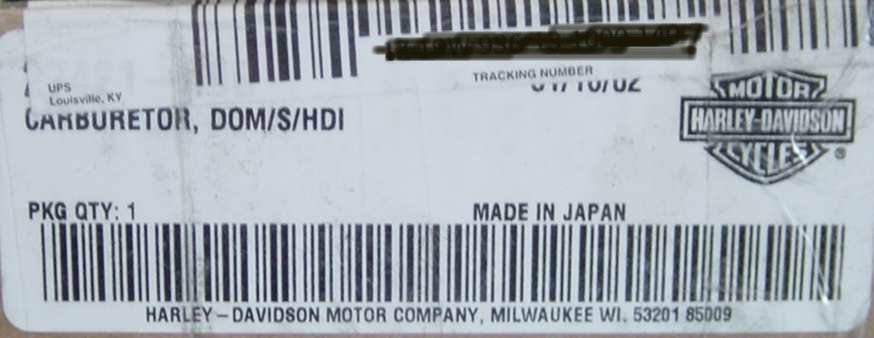The photograph features a weathered and slightly dirty barcode label affiliated with Harley-Davidson Motorcycles. The label, which has transparent tape affixed to a box, prominently displays several key details. In the top right corner, the Harley-Davidson Motorcycles logo stands out. Below it, the label reads "Motor Harley-Davidson Cycles." 

In the upper section, there is a standard barcode with thick and thin black lines. Directly beneath the barcode, a black marker has been used to cross out a tracking number, followed by the words "tracking number." 

To the left, the label reads "Carburetor DOM/S/HDI," and beneath this, "Made in Japan" is indicated. The lower part of the label specifies the package details, stating "Package Quantity: 1." Additionally, the label includes the address, "Harley-Davidson Motor Company, Milwaukee, Wisconsin 53201-8500." Overall, the label appears slightly worn, signifying it has been through some rough handling.